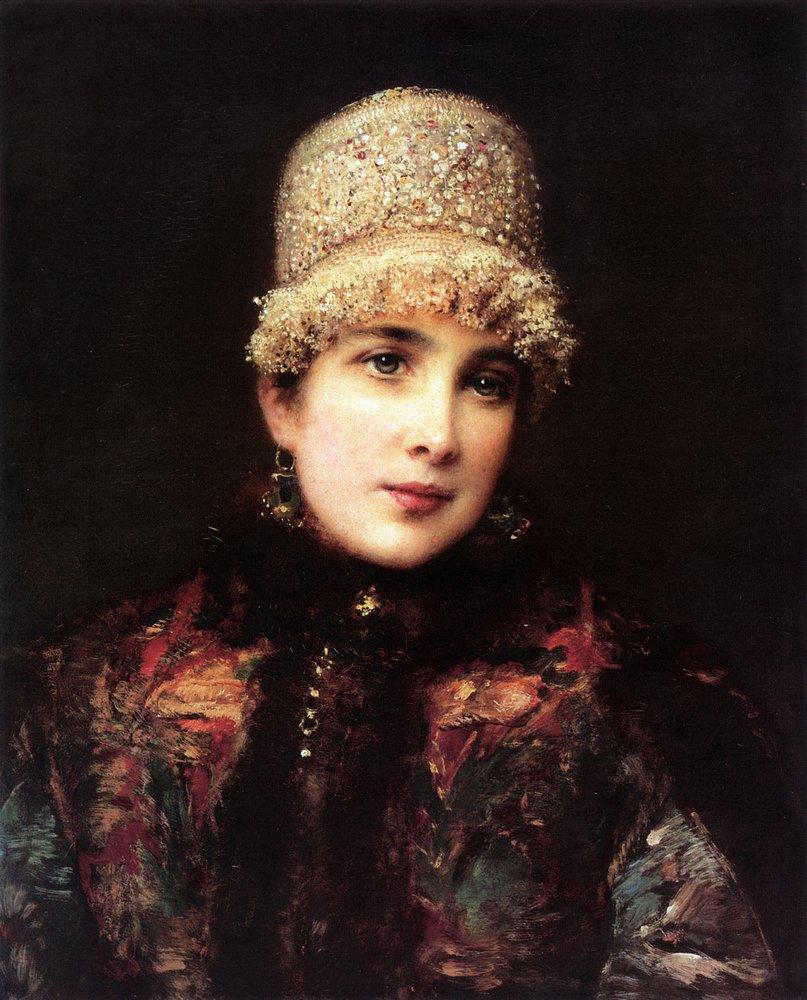In this highly detailed and elegant painting, a woman in her 20s or 30s with a very fair, milky pale complexion and striking blue eyes gazes off to her left against a solid black background. She wears vibrant dark red lipstick, and her look is accentuated by large, dangling hoop earrings. Atop her head, she dons a tan bucket hat adorned with white and red sequins, and a fuzzy rim that suggests a plush texture. The woman is wrapped in a luxurious, eye-catching, multicolored jacket that exudes richness and elegance, resembling a mink coat with an intricate floral pattern woven in dark brown, red, beige, and lighter blue colors. The coat, featuring feathery textures around the chest and arms and a black woolly collar, further enhances her opulent appearance. The painter’s skillful rendering gives this artwork a lifelike realism that blurs the line between painting and photograph.